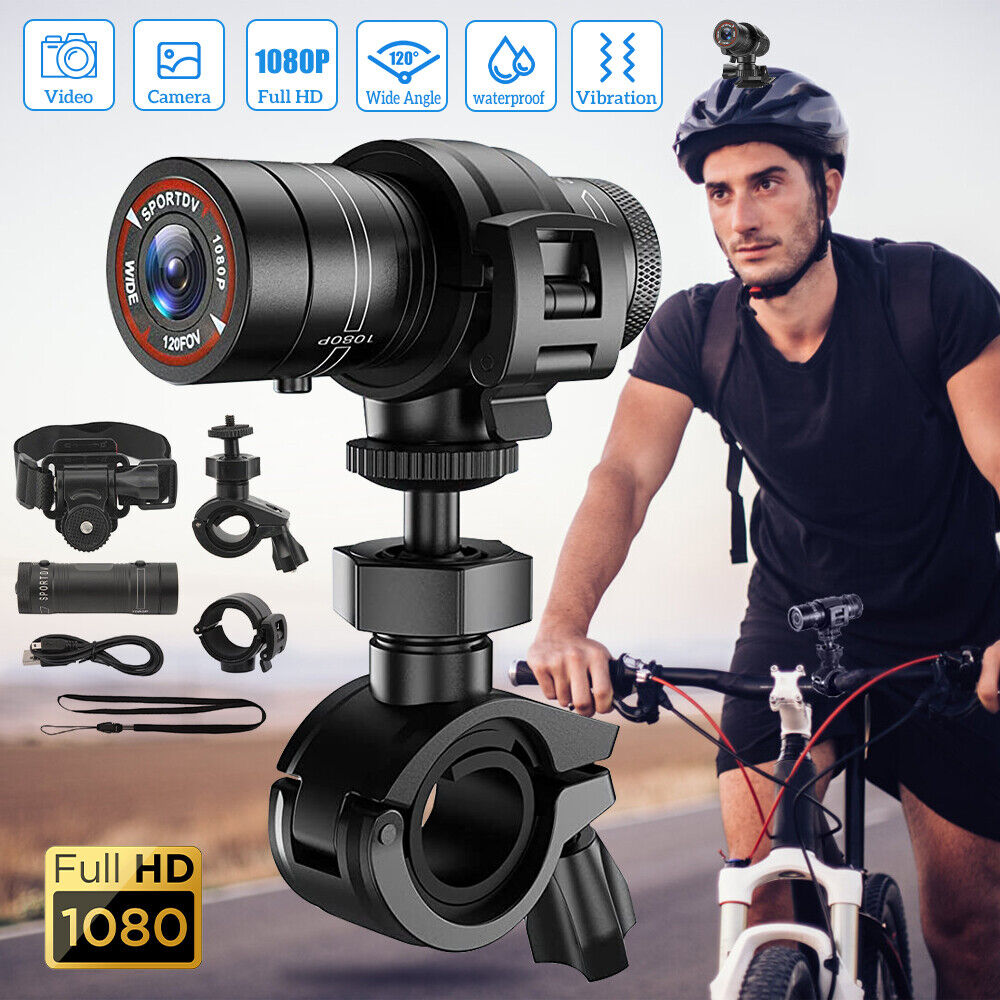The image is a detailed promotional advertisement for a Sport DV camera designed to be mounted on bicycles. On the right side, a man wearing a blue outfit, including a helmet, rides a white-framed bicycle with black handlebars. The camera is shown attached to both the helmet and the bike's handlebars, although these cameras appear to be digitally imposed. To the left, there is a close-up of the camera accompanied by numerous accessories like clamps and cords, floating around it. In the upper left corner, several white square icons highlight the camera's features, stating "video," "camera," "1080p full HD," "120 wide-angle," "waterproof," and "vibration." Additionally, a gold box in the bottom left corner prominently displays "Full HD 1080." This comprehensive layout emphasizes the camera's multifunctionality and high-definition capabilities, making it a suitable tool for capturing biking adventures.